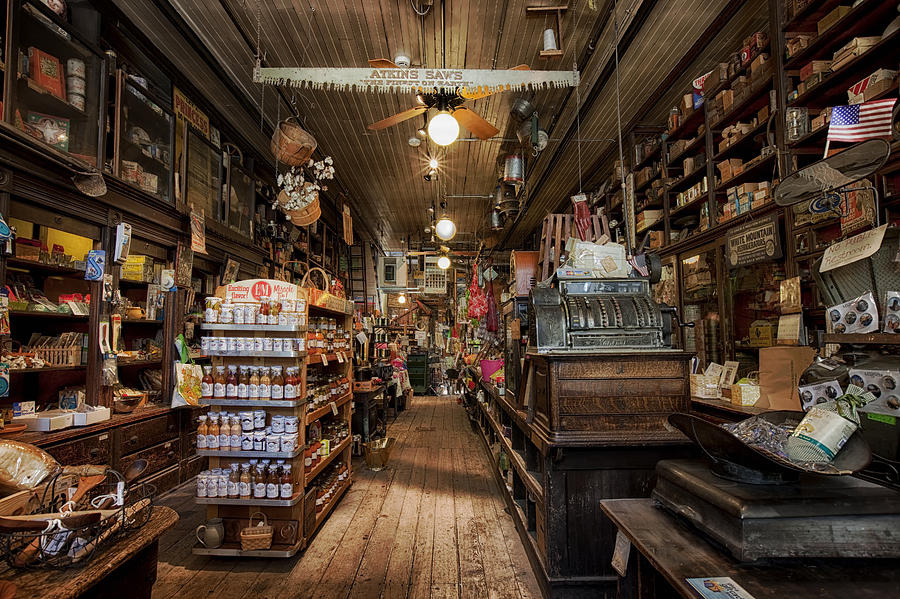This image captures the interior of an old-time, vintage general store with a rich historical ambiance. The ceiling and floor are composed of dark wood planks, complementing the overall rustic aesthetic. Suspended from the ceiling are multiple lights, a ceiling fan, and a notable saw blade emblazoned with "Atkins Saws." On both sides of the store are wooden shelves brimming with a variety of items, contributing to an eclectic and stocked environment. Particularly in the center, a prominent shelf displays an array of spices and seasonings, while to the right, a metal cash register sits on a wooden counter, enhancing the nostalgic appeal. Additionally, jars of homemade items like jams, jellies, and sauces can be seen, further adding to the old-fashioned charm of this space that feels like a genuine walk through history.